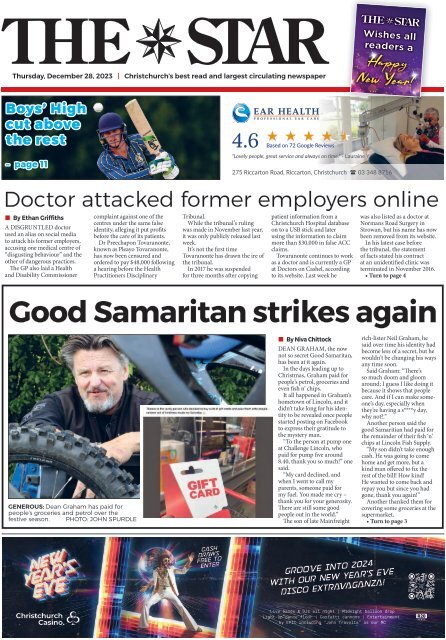The image depicts a newspaper article displayed on a website with a prominent white background. At the top, the title "THE STAR" is presented in capital letters and bold black font, with a 3D star graphic situated between the words. To the right, there is a rectangular purple banner with the phrase "The Star Wishes You a Happy New Year!" in bold yellow text at the bottom, set against a top section in white.

Below this, on the left, the date is listed as "Thursday, December 28th, 2023." The newspaper is identified as "Christ Church's Best Read and Largest Circulating Newspaper," though the text is somewhat blurry. A red line spans across the page, separating different sections.

One headline, outlined in blue, reads "Why A Boy's High Cut Above The Rest" on page 11. On the right side, the phrase "Air Health" is displayed in blue text, accompanied by a 4.6-star rating icon. Another headline in black states, "Doctor Attacked Former Employers Online."

Towards the bottom, inside a black-outlined box, the title "Good Samaritan Strikes Again" appears in bold letters, accompanied by an image of a man with a tire in front of him. Upon zooming in, the caption reveals that the man, identified as Dean Graham, has paid for people's groceries and fuel, though the remaining details of the text are unclear.